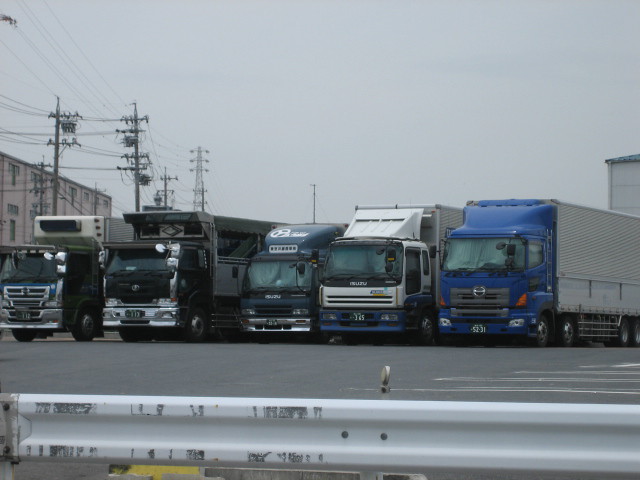The image depicts a dreary, overcast day outside with a gray sky, devoid of any sunlight. Dominating the left side is a tall business-like building, accompanied by several telephone poles brimming with wires. The center of the image features a spacious parking lot outlined with parking lines. In the foreground, there's a stainless steel or gray guardrail.

In the parking lot, five mid-sized trucks are parked in a row, varying slightly in size but generally smaller than standard 18-wheelers. Starting from the left, the first two trucks have silver bumpers and grilles, the third boasts a blue front with a silver bumper, the fourth presents a blue bumper with a white body, and the fifth includes a gray grille with a body fully painted in blue. Each truck has a white bed, except the middle one, which is smaller and painted a dark greenish-blue color. Additionally, the first truck features a large blue front, and behind it sits a warehouse-style building. Scattered across the background are more buildings and larger telephone poles, adding to the industrial atmosphere of the scene.